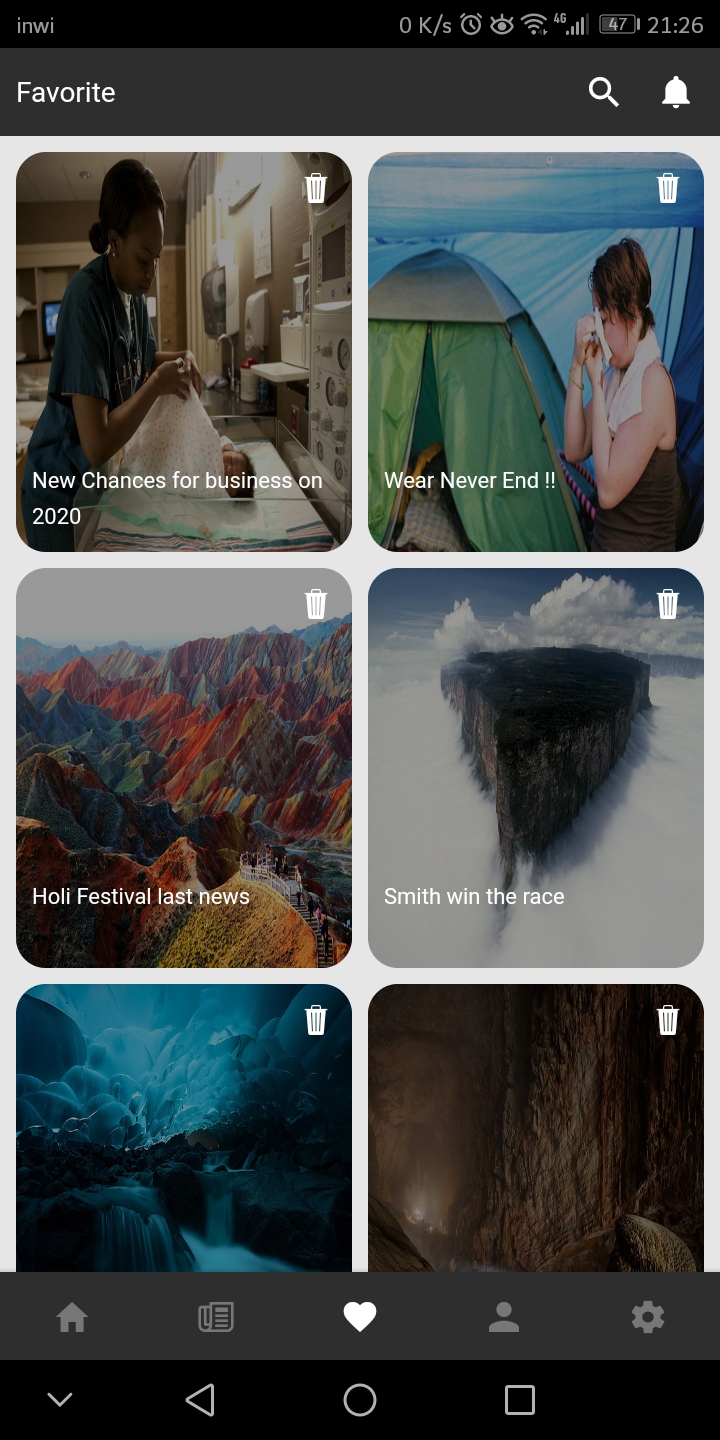This image is a detailed screenshot taken on a smartphone. The app in use is unclear, but in the top-left corner, partial app initials "R-I-N-W-I" are visible. Standard phone icons are present at the top of the screen, which include an alarm indicator, reflecting the time set to 21:26, possibly in military time. 

The primary screen content is a gray interface featuring the word "Favorites" at the top, accompanied by a magnifying glass icon for search functionalities and a bell icon for notifications. The main interface displays a series of tiles, each equipped with a delete button in the top right corner, and a title along with an associated image in the lower left corner.

One tile features a photo of a Black woman who appears to be either sewing or unpacking items from plastic bags, with the caption "New chances for business on 2020," and suggests a home environment. Another tile, captioned "Wear never ends," shows an Asian woman amidst a camping scene with two tents visible in the background.

A further tile reads "Holly Festival latest news," depicting a vividly colorful mountain range. Another tile, titled "Smith wins the race," shows a solitary mountain peak cloaked in clouds. Additional tiles are present but not fully visible in the screenshot.